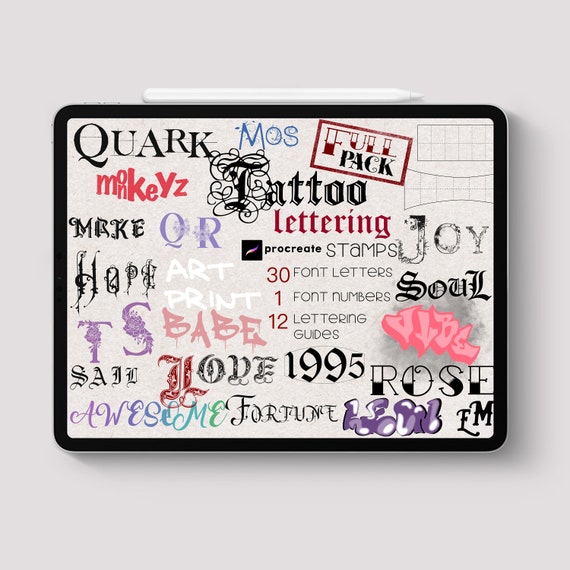The image depicts an aerial view of an iPad with an Apple Pencil magnetically attached to the top. It lies against a gray-white background. The iPad screen displays a Procreate app open to a collage of various font names, including Quark, Mouse, Monkeys with a Z, Tattoo, Lettering, Full Pack, Joy, Soul, Vibe, and Rose. Each font name visually portrays its respective style—such as the medieval-themed Tattoo Lettering and the graffiti-inspired Vibe. Additionally, the text on the screen mentions "Procreate stamps," indicating that this is a pack for sale containing 30 font letters, 1 set of numbers, and 12 lettering guides, catering to users of the Procreate drawing program for iOS.